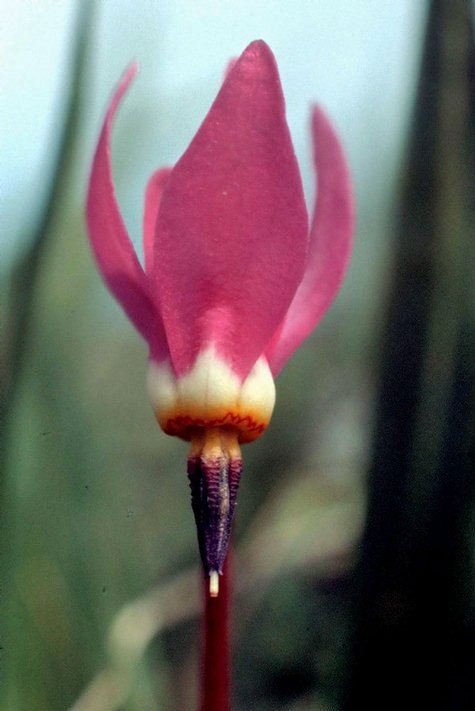A detailed, descriptive caption for the image could be:

---

This photograph features an extreme close-up of a flower, intensely focused on the bloom while the background is rendered into a soft, abstract blur of greens, blues, and whites, reminiscent of out-of-focus foliage. The entire image carries a grainy texture, peppered with specks of grungy artifacts, suggesting either intentional artistic enhancements or imperfections from the image capture process.

The flower, dominating the entire frame, exhibits unopened petals that rise sharply in a bulb-like formation. There are approximately four or five distinguishable petals, with noticeable gaps between them, hinting that some petals might be hidden or yet to unfurl. The petals create a layered effect with one central petal flanked by one to the left, one to the right, and two partially visible behind.

At the base of the petals, the flower displays a striking color gradient: starting with a delicate white at the flower's core, transitioning through shades of yellow and orange, and culminating in a vivid red where it meets the stem. The stem itself appears unusual with a cluster of elements at the base, possibly buds or leaves, adding to the complex beauty of the plant. The overall composition, though detailed and colorful, retains a dreamy and somewhat mysterious aura due to the blurriness and graininess of the image.